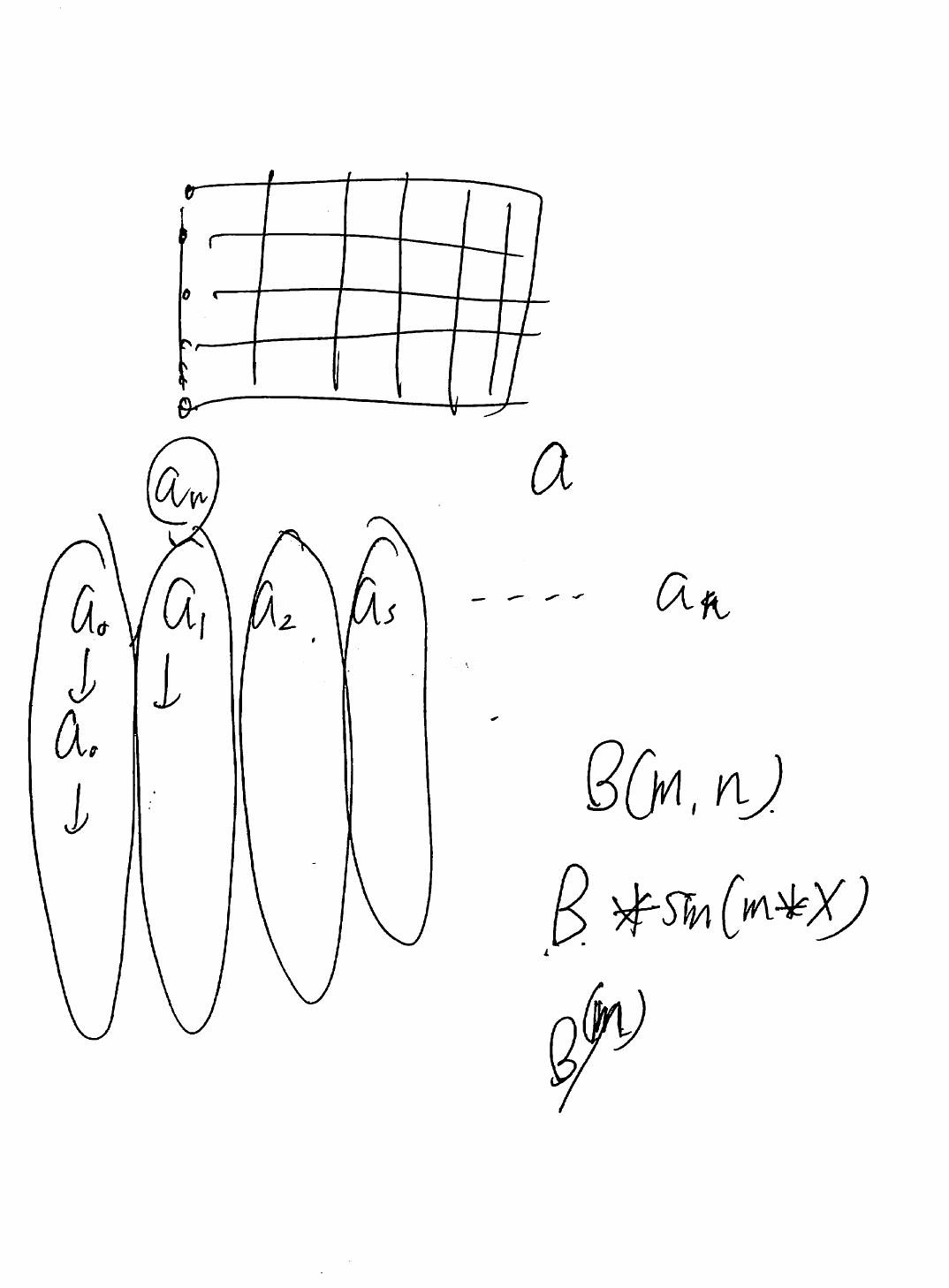The image depicts a meticulously crafted black ink drawing on a pristine white background. The composition is dominated by a large, somewhat messy rectangular shape at the top, featuring an intricate grid of vertical and horizontal lines that are incomplete in their traversal, giving a fragmented appearance. Along the left edge of the rectangle, there are eight circles. The first four circles are evenly spaced and align with the horizontal lines of the grid, whereas the last three circles are clustered closer together.

Further detailing reveals a series of elongated, vertical ovals containing various letters and symbols interspersed within this system of lines and circles. Notably, there are dots accompanied by arrows pointing downward, which suggest a sequence or flow. For instance, there is a dot with a downward arrow followed by another combination where a circle tops an elongated vertical oval marked "A-N." Additional annotations within the ovals include labels like "A-1" with an arrow pointing downwards, "A-2," "A-S," and a repeated "A-N." The sequence continues with distinctive symbols such as "B" with an asterisk and abbreviations "S" and "M," suggesting specific meanings or functions within the overall structure.

The careful placement of these elements and the deliberate use of symbolic notation imbues the drawing with a sense of technical or diagrammatic precision, evoking the essence of an abstract schematic or conceptual map.